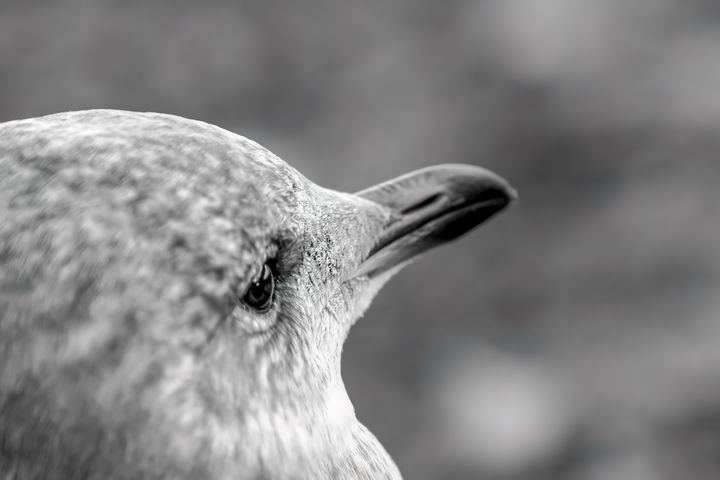In this striking black and white photograph, the blurred background appears to be taken outdoors, possibly in a natural environment such as a valley or among trees, given the various shades of gray ranging from dark to light. Dominating the center of the image is a close-up of a bird's head, specifically its right side. The bird’s smooth, silky feathers display shades of gray and white, giving it a fur-like texture that almost resembles that of a dog. The upper portion of the bird is depicted with a clear, bright eye, and a long, pointed beak, which is subtly highlighted by the small hole near its nasal area. The bird is captured looking up towards the upper right corner of the frame, lending an impression that it is observing something intriguing in the distance. The focus on the bird’s eye and beak, coupled with the soft, blurred background, creates a compelling sense of depth and detail in this photograph.